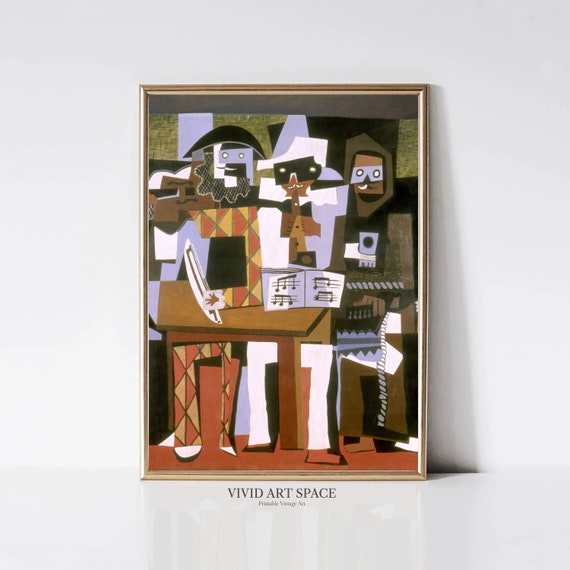This image captures an intriguing, abstract art piece named "Vivid Art Space." Set against a grey background with a slight grey strip at the top, the artwork is encased in a gold frame resting on a white countertop. The art itself prominently features three human-like figures composed of various geometric shapes and vibrant colors. Each figure has distinct square or rectangular heads with rectangular overlays resembling masks over their eyes, embellished with beady, round eyes. The person on the left is dressed in a suit with a diamond pattern of red and yellow, wears a black hat, and sports a black beard. This character holds what appears to be a violin bow in their left hand, although the instrument is partially obscured. Central to the composition is a figure with black glasses holding a sheet music book, highlighted by its musical notes. The character on the right dons a brown hood and pants adorned with patterns that resemble keyboards, and holds a brown object that could be interpreted as a gun. Dominating the right-center of the image is a brown wooden table adding a tangible element to the whimsical scene. The figures, rendered in a cartoonish, almost disjointed style, seem to interact with the elements around them, creating a dynamic and enigmatic visual narrative. At the bottom of the grey strip beneath the frame, the title "Vivid Art Space" is inscribed, with smaller text that adds a finishing touch to the detailed, multi-layered composition.